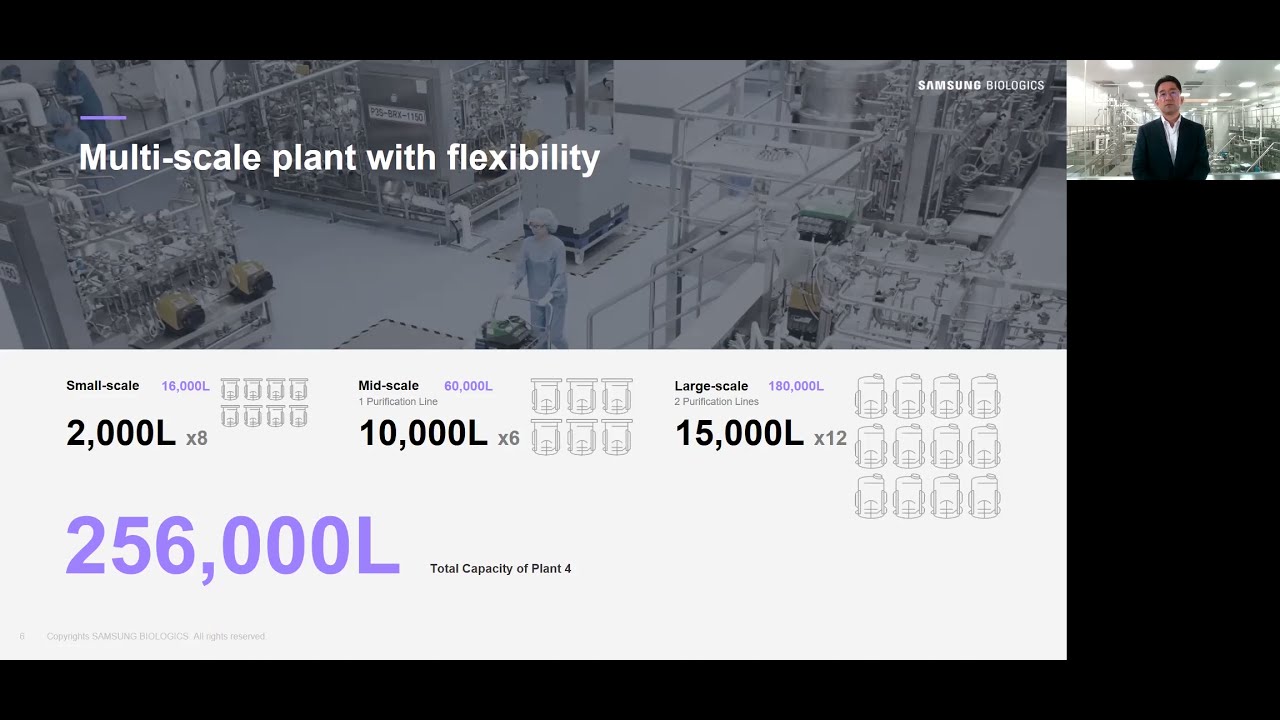The image appears to be an advertisement by Samsung Biologics, presented in an aerial, sans-serif white font that reads "Multi-Scale Plant with Flexibility." The backdrop of the image seems faded and gray, almost like a blueprint or a photo, with a few distinct visual elements. 

In the top right corner, there's the Samsung logo with the word "Biologics" next to it. Below this, there’s a picture of an Asian male wearing a business suit and a white-collared shirt standing in front of what looks like a factory or warehouse. 

Centered within the image is another scene showing what looks like a person in scrubs and a hair mask, possibly pushing a cart inside the factory. Overlaying this part of the image is text in white font describing the plant's capacity in different scales: 

- **Small scale:** 2,000L x 8, equaling 16,000L
- **Mid scale:** 10,000L x 6, equaling 60,000L, with 1 purification line
- **Large scale:** 15,000L x 12, equaling 180,000L, with 2 purification lines

At the bottom, a light lavender-colored font states the "Total capacity of Plant 4" as 256,000L. This advertisement aims to showcase Samsung Biologics' extensive and flexible manufacturing capabilities across various scales, emphasizing their ability to support a wide range of biological production needs.